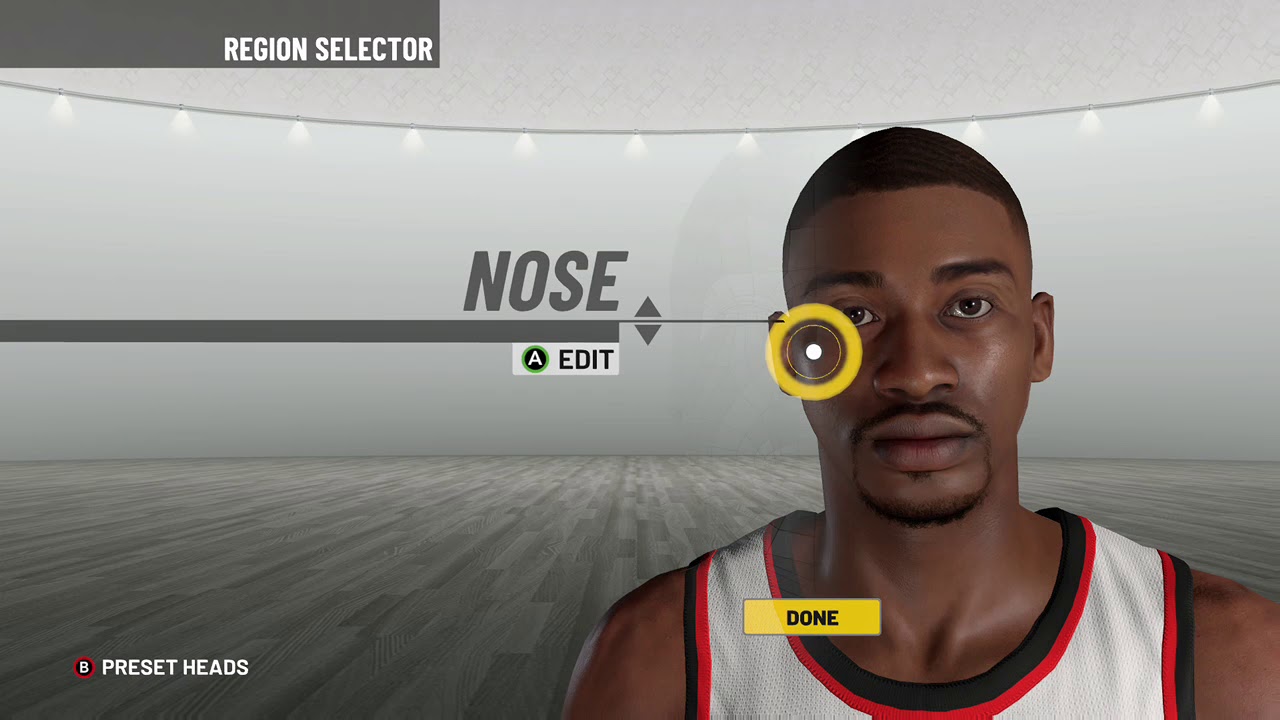The image appears to be a screenshot from a basketball video game, specifically from a character creation screen. The central focus is on a male character visible from the shoulders up, wearing a predominantly white jersey with black and red accents. He has a beard and mustache, and a distinguishing yellow ring on his face. On the left side of the screen, "NOSE" is displayed in bold, grey letters above a grey line, accompanied by an "A" within a green and black circle, followed by the word "EDIT" in black. Up and down arrows are positioned next to "NOSE," indicating that these controls can be used to adjust the character's nose. The background depicts an empty, white room with tiled flooring and rounded walls, illuminated by overhead lights. Below the character's image, the word "DONE" is visible, while "PRESET HEADS" is located in the bottom left corner. Additionally, the phrase "REGION SELECTOR" is situated in the upper left corner of the screen.